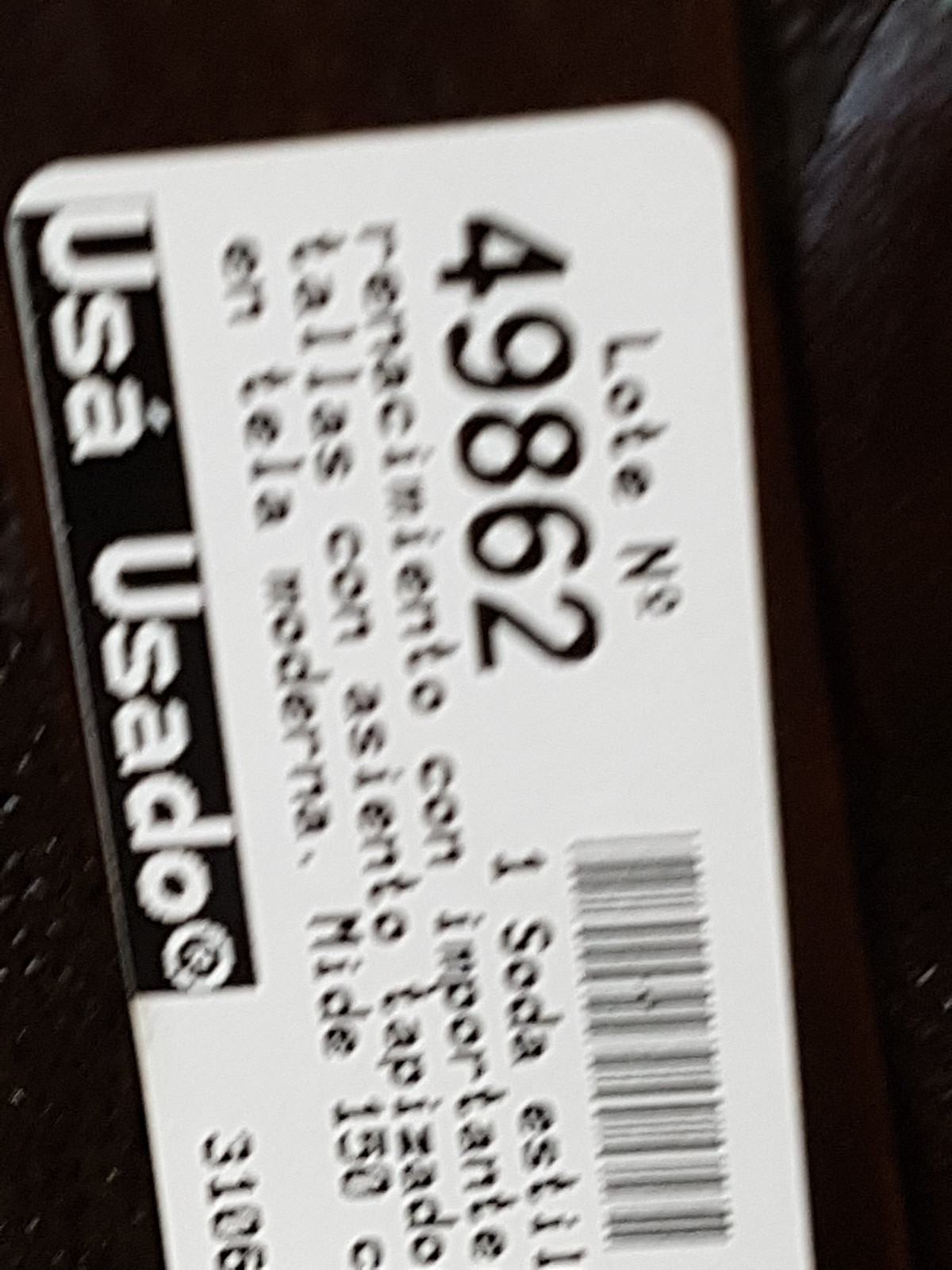This image features a close-up of a white rectangular label with rounded corners, positioned on a piece of brown leather, possibly a sofa chair. The label, which is vertically oriented within the frame, is slightly tilted so that the left side appears at the top of the image. The text on the label is primarily in Spanish and includes "lote número 49-862" prominently displayed in black. Below the lot number, there's a barcode followed by several lines of text in smaller font, which are partially obscured and blurry. The visible text includes phrases like "uno soda estilo renacimiento con importante" and "talles de con asiento tapacido," though some words are missing or unclear. The label also features a small black banner with white text at the bottom left corner that repeats "USA USADO."